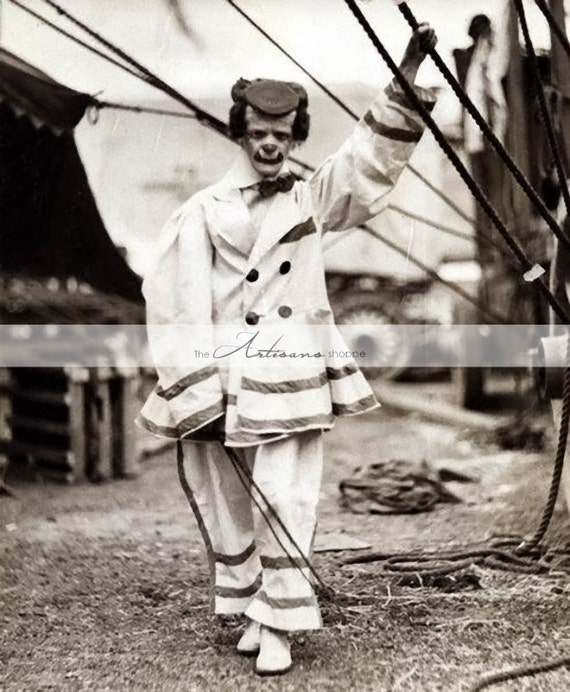This vertical, black-and-white photograph, likely taken over a century ago, evokes an eerie atmosphere with its portrayal of a clown on a grassy and dirt-covered ground. The clown, dressed in a baggy, oversized white suit with distinct stripes along the bottom of the jacket and pants, and large buttons down the front, walks toward the viewer with an ominous expression. His white shoes and a small, round hat add to his disconcerting appearance, bolstered by heavy, unnatural-looking makeup accentuating his eyes, nose, and mouth. His left arm is stretched above him, gripping a dark-colored rope that contributes to a makeshift fence, while his right hand holds some sort of stick. Bushy, dark hair peeks out from under his hat. Blurry in the backdrop is a large tank viewed from the side, featuring a large wheel partially covered by canvas. The top part of the image is a sky that appears white and brown. The photograph is unsettling, with the clown's emaciated form contrasting sharply with his voluminous attire, creating a lasting impression of creepiness and unease.